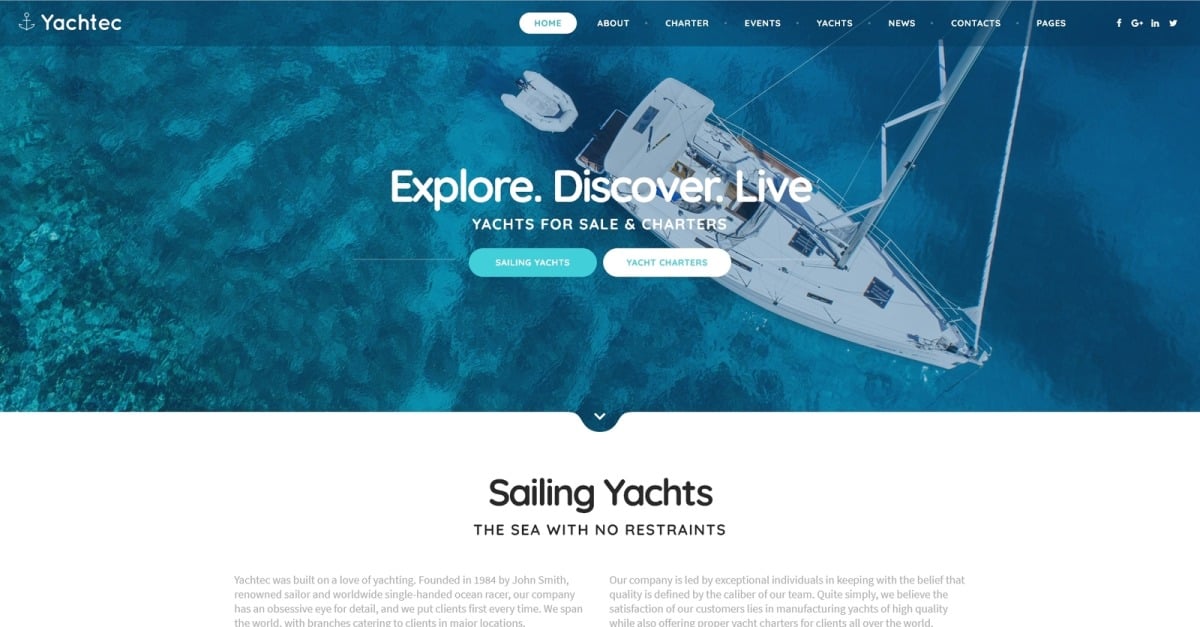**Caption:**

A luxurious yacht floats gracefully on the clear, multi-shaded blue waters. The vessel, equipped with railings and a visible sail bar (currently without a sail), features a back platform for passengers to stand on and relax. A small speedboat is being towed behind it, enhancing the allure of maritime adventure. 

Above the image, a dark blue navigation bar features the logo "Yacht Tech" accompanied by an anchor symbol. This bar includes menu items such as Home, About, Charter, Events, Yachts, News, Contacts, and Pages, alongside icons for social media platforms like Facebook, Google+, LinkedIn, and Twitter (now X). 

Bold white text across the water proclaims, "Explore, Discover, Live. Yachts for Sale and Charters. Sailing Yachts and Yacht Charters." Two buttons, one blue and one white, invite users to click for more information, ensuring an immersive online experience for sailing enthusiasts.